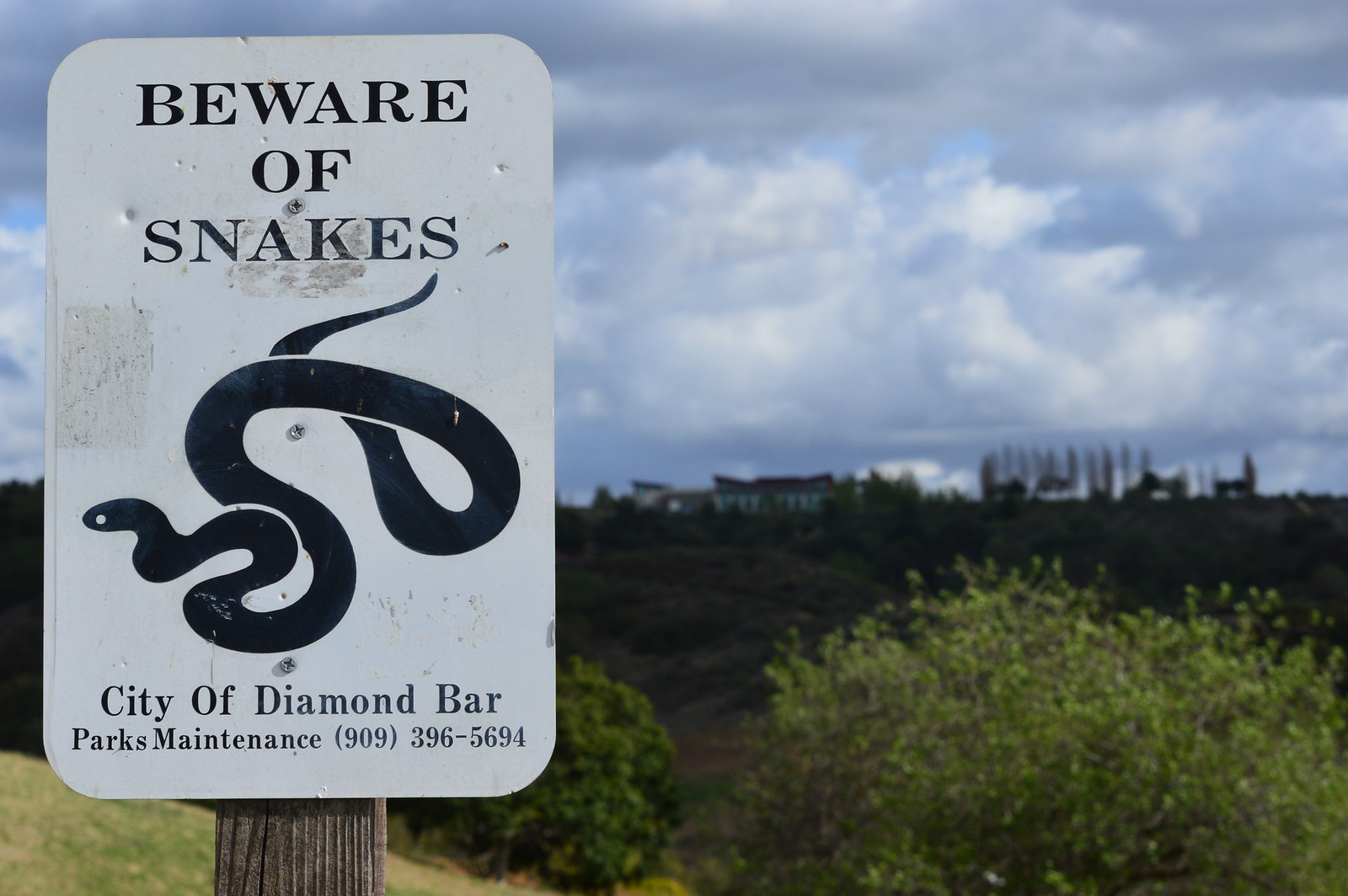This photograph captures a close-up view of a rectangular white warning sign attached to a brown wooden pole, located in an outdoor setting. The sign, which is the main focal point and is secured with screws to the pole, cautions with the text "BEWARE OF SNAKES" written in bold black capital letters at the top. Below this warning, there is a detailed black drawing of a coiled snake facing left. Further down, the sign lists "City of Diamond Bar, Parks Maintenance" followed by the phone number "909-396-5694" in black font. 

In the background of the image, which is primarily on the right side and slightly out of focus, there is uneven ground covered with plants and grass, as well as green rolling hills adorned with various bushes and trees. Above the landscape, the sky appears mostly filled with white and gray puffy clouds, suggesting an overcast day with the sun obscured, casting a dim light over the scene. The horizon in the background hints at a distant building and possibly some motor vehicles amidst the natural setting.